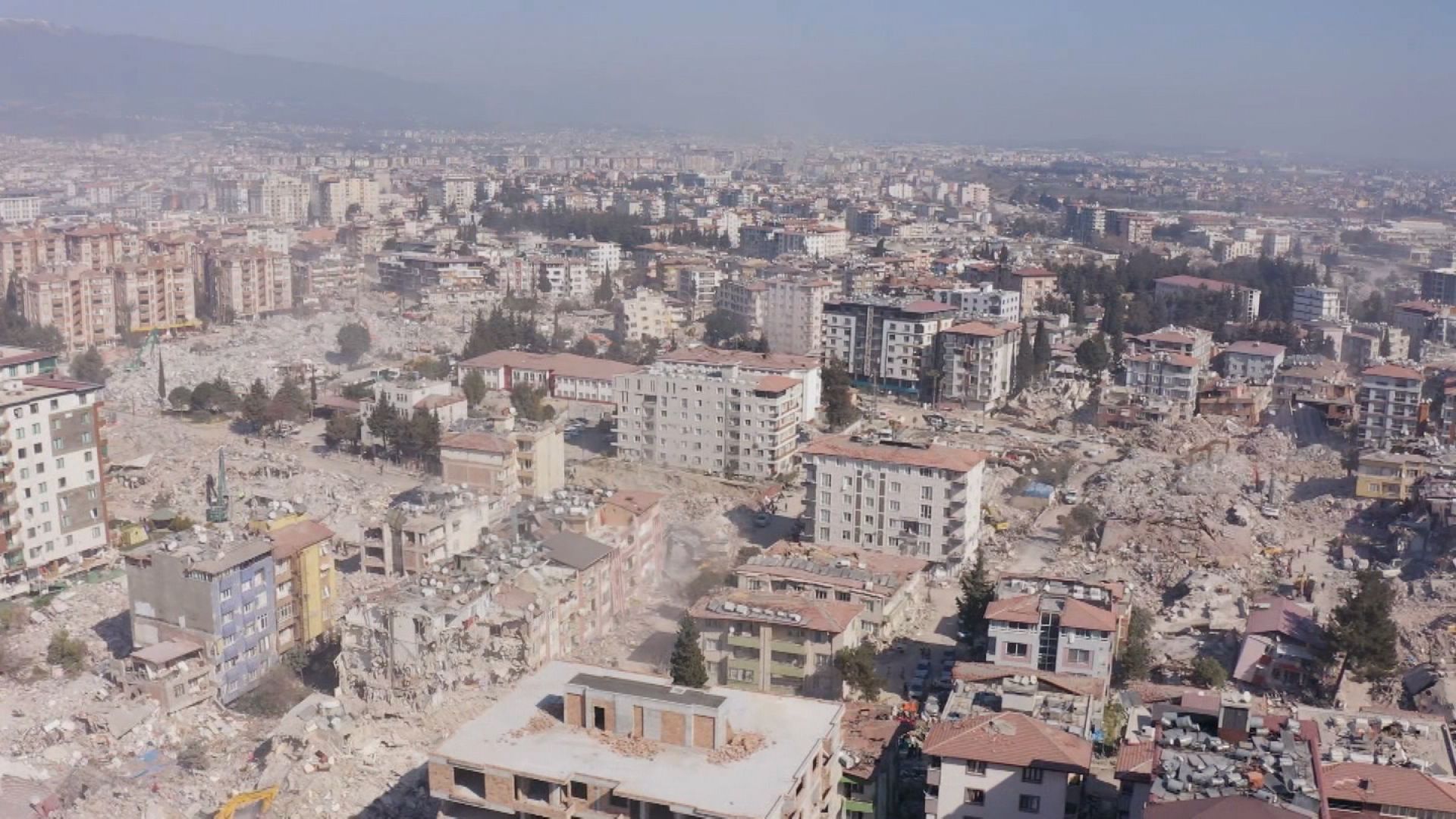The aerial photograph, likely taken by a drone, captures the devastating aftermath of a massive earthquake that struck Turkey in February 2023, as reported by CNN. The image presents a city, once bustling and vibrant, now marred by destruction and rubble. Pockets of debris are visible throughout, with some buildings completely reduced to piles of bricks and dust. The structural chaos is more concentrated in the bottom center, bottom left, and right sections of the photo, where multi-story buildings lie in ruins.

Amidst the devastation, numerous buildings still stand, albeit in various states of disrepair. Some structures have their roofs caved in, while others retain their maroon-colored or white roofs. The remaining facades are mostly beige, and the buildings range from eight to ten stories tall. Despite the severe damage, the original urban layout is discernible, revealing a densely built city that formerly housed thousands of structures.

The upper part of the image shows the city sprawling into the horizon, emphasizing the extensive reach of the calamity. A foggy or slate-colored sky looms overhead, contributing to the somber tone of the scene. A mountain peak is visible on the horizon in the upper left, punctuating the landscape.

Absent from the photograph are the ongoing rescue efforts, leaving the viewer to focus solely on the scale of destruction. The sheer magnitude of the damage—encompassing dozens of collapsed buildings and countless others in compromised conditions—paints a stark picture of the disaster's impact.